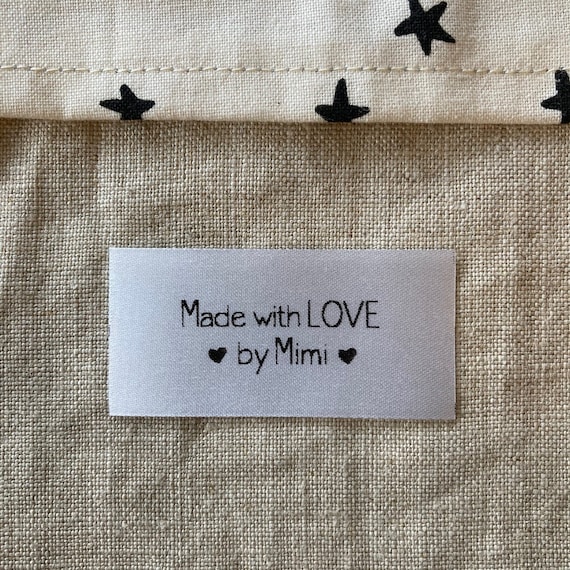The photograph is a close-up of a handcrafted item made from a burlap-like material, likely a heavy linen in earthy tones of light tan, beige, and brown. The object, which might be a bag or garment, features distinct stitching and black star patterns across the top lighter tan part. Central to the image is a white label with black text that reads "Made With Love by Mimi," flanked by two black heart symbols on either side of "Mimi." The combination of the earthy hues, detailed stitching, and personalized label suggests a handmade, possibly artisanal product.